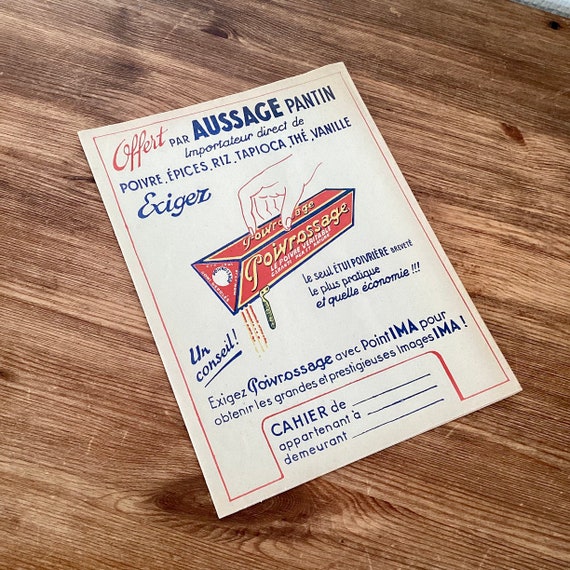This image showcases an old flyer, likely from the 1970s, weathered and printed on pale brown parchment. The flyer lies on a medium-toned, slightly worn wooden table. Prominently featured on the flyer is a woman's cartoon-style hand holding a red package, which might be cookies or crackers, and this package is adorned with yellow lettering that reads "P-O-W-R-O-S-S-A-G-E." The top of the flyer bears the heading "Offert" in red, followed by “Au Faire Poissuage Pantin, Imporator Direct de Poivre, Épices Riz Tapioca, Thé Vanille” in blue. Additionally, the flyer includes French text throughout, notably "Cahiers d'appartements et d'amirants" situated at the bottom. The combination of the vintage aesthetic and the detailed French text suggests an advertising poster from a bygone era.